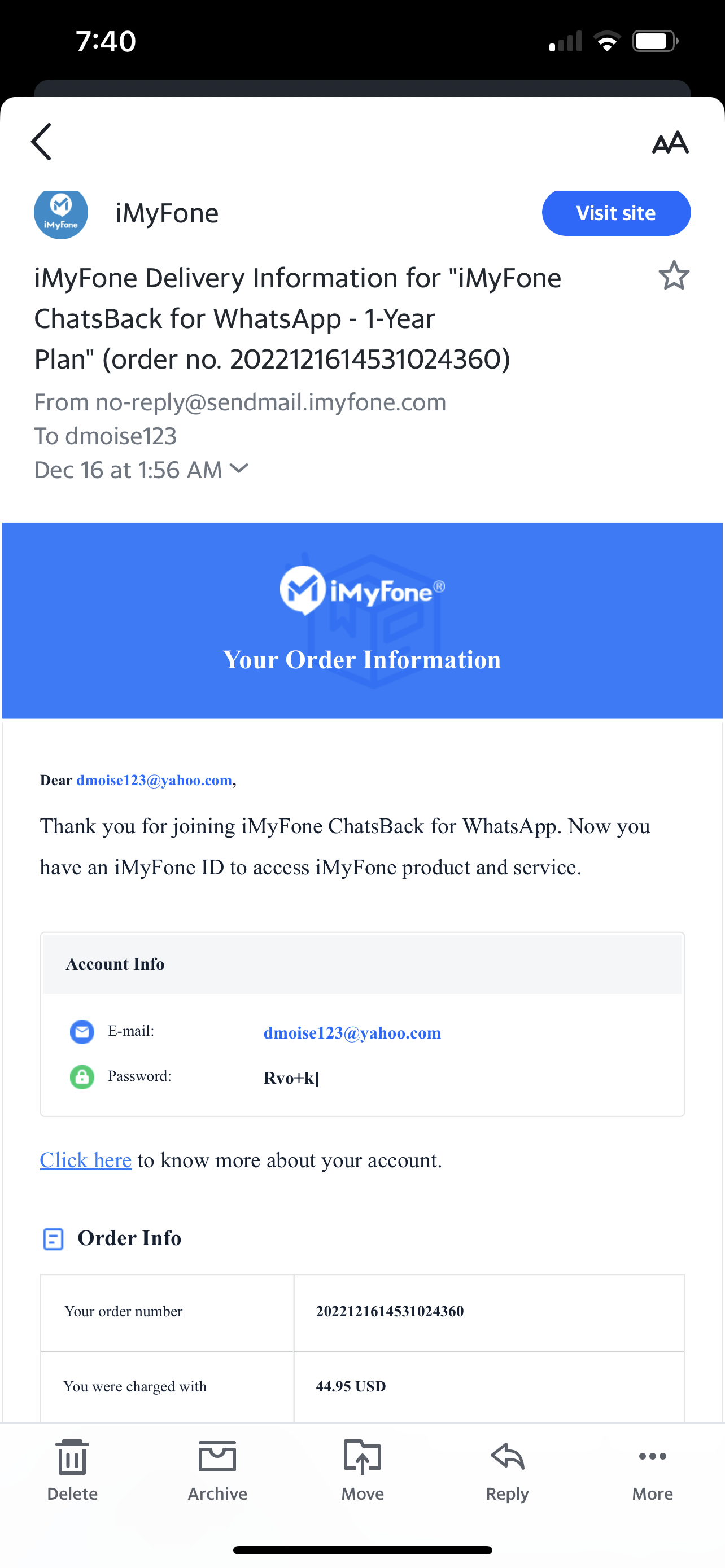This image is a vertical screenshot taken from a cell phone. At the top of the screen, a black bar displays the time "7:40" in white text on the upper left corner, alongside icons for battery status and Wi-Fi signal on the upper right. Below this black bar, the background is predominantly white with black text throughout.

The main section begins with a blue circular icon containing a white "M" to the left of the text "iMyFone", which also appears again directly below the icon. To the right of the "iMyFone" text, there is a blue, clickable oval button labeled "Visit Site".

Further down, the text "iMyFone delivery information for iMyFone ChatsBack for WhatsApp-1-year plan, order number" is followed by a long numerical sequence. The sender information reads: "From: no-reply@sendmail.imyfone.com To: D Mois, 123 Date: December 16th at 1:56 AM".

Approximately a third of the way down the image, there is a prominent blue rectangle featuring the same "iMyFone" circular icon with the white "M". Inside this box, it says "iMyFone Your Order Information".

Beneath this blue box, a white section with black text begins with a greeting: "Dear D Mois, 123 at yahoo.com, Thank you for joining iMyFone ChatsBack for WhatsApp. Now you have an iMyFone ID to access iMyFone products and services. Account info Email: D Mois, 123 at yahoo.com Password: RBO plus K something." Following this is a blue, underlined link labeled "click here" to know more about the account.

An "Order Info" section follows, listing the order number again with the same lengthy numeric sequence, and it states a charge of $44.95 USD.

At the bottom of the screenshot, visible icons for actions such as delete, archive, move, reply, and more are displayed.